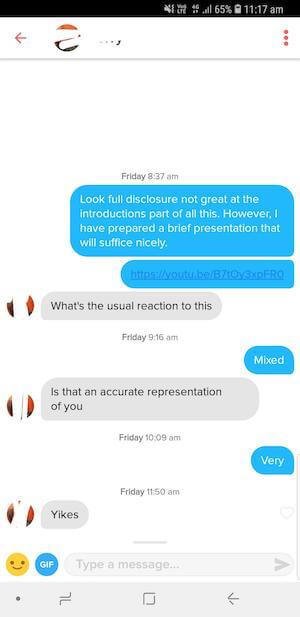The image showcases a series of screenshots from a messaging app conversation. Dominating the upper section of the screenshots is a black status bar that displays multiple icons: a muted microphone, voice over LTE (VoLTE), network signal strength showing 25 out of 5 bars, a battery level at 65%, and the time, 11:17 AM. Beneath the status bar, a timestamp is visible indicating "Friday 8:17 AM," followed by a message that reads, "Look, full disclosure, I’m not great at the introductions part of all this. However, I have prepared a brief presentation that will suffice nicely. Here's a link given."

The conversation continues with the other person asking, "What's the usual reaction to this?" To which the first person responds, "Mixed." The second person then queries, "Is that an accurate representation of you?" The first person succinctly replies, "Very." The final response in the sequence is a single word, "Yikes," signaling an apparent disfavor towards the initial message and link.

At the bottom of the screenshots, the standard navigation keys for recent apps, home, and back are clearly visible, marking the familiar interface of many smartphones. This detailed visual provides insight into the nuanced exchanges typical within messaging apps, capturing both the conversation and the device interface.